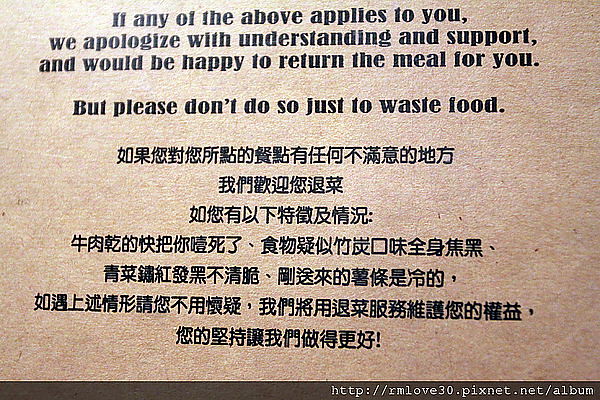The image is of a sign, seemingly painted or printed onto a light brown wall, which transitions to a darker brown shade near the base, likely due to a ceiling light source. The sign features a bilingual message, with four lines of black text in English at the top and six lines of text in Chinese or Japanese script below. The English text reads, "If any of the above applies to you, we apologize with understanding and support and would be happy to return the meal for you. But please don't do so just to waste food." Below the bilingual text, there is a dark brown strip containing a web address: rmlove30.pixnet.net. This sign serves as an announcement discouraging the waste of food.